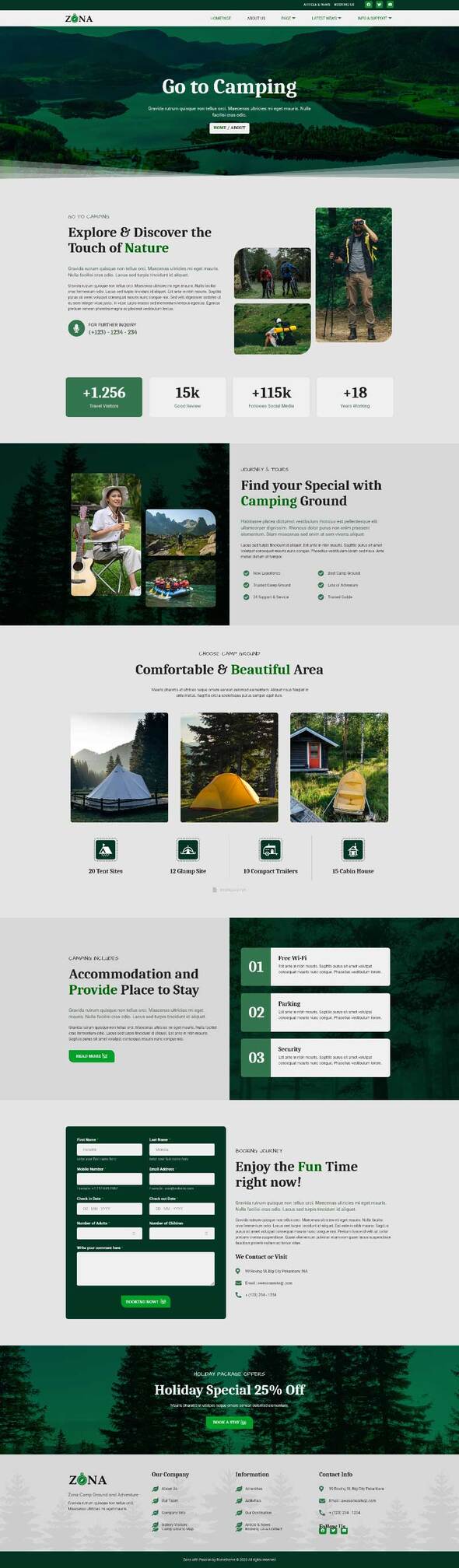This screenshot exhibits a desktop website mockup, possibly titled "Zona," displayed on an unspecified browser and operating system. The image quality is notably poor – small and blurry – making some details hard to decipher. However, some elements can still be distinguished.

The top section features a dark green navigation bar packed with various social media icons such as Facebook, Twitter, and email, though the exact labels are unreadable. Below, there is a white navigation bar presenting several options, including "About Us," "Latest News," "Info and Support," and other indistinct texts.

Central to the design is a visually filtered image of a lake, accompanied by the text “Go to camping” followed by placeholder Latin text. A prominent rectangular box below displays breadcrumbs reading “Home / Account” and additional phrases like “Go to camping” and “Explore and discover the touch of nature,” interspersed with more Latin filler text. Noteworthy statistics are also featured: 1.256 (visitors), 15K (social media followers), 115K+ (reviews), and a figure of 18, though their exact contexts are indiscernible.

Further down, the site exhibits various camping photos with labels such as "Journey and Tours" and "Find your special camping ground," along with descriptive texts. The subsequent section outlines "Choose Campground," showcasing options such as 20 tent sites, 12 glamp sites, 10 compact trailers, and 15 cabin houses, emphasizing comfortable and beautiful camping areas.

Additionally, the “Camping Includes” segment suggests the inclusion of accommodation amenities, with links to read more details (text is Latin placeholder). Adjacent to this is information on facilities like free Wi-Fi, parking, and security. There's also a form inviting visitors to book their journey with text that prompts “Enjoy the fun times right now.”

Promotional offers are highlighted next, particularly a holiday special with a 25% discount. Lastly, the website footer appears to house contact information and company details, although these sections also contain placeholder text.

This comprehensive layout suggests the site is designed for a camping service provider, potentially still in the development or revision stages due to the prevalence of placeholder content.